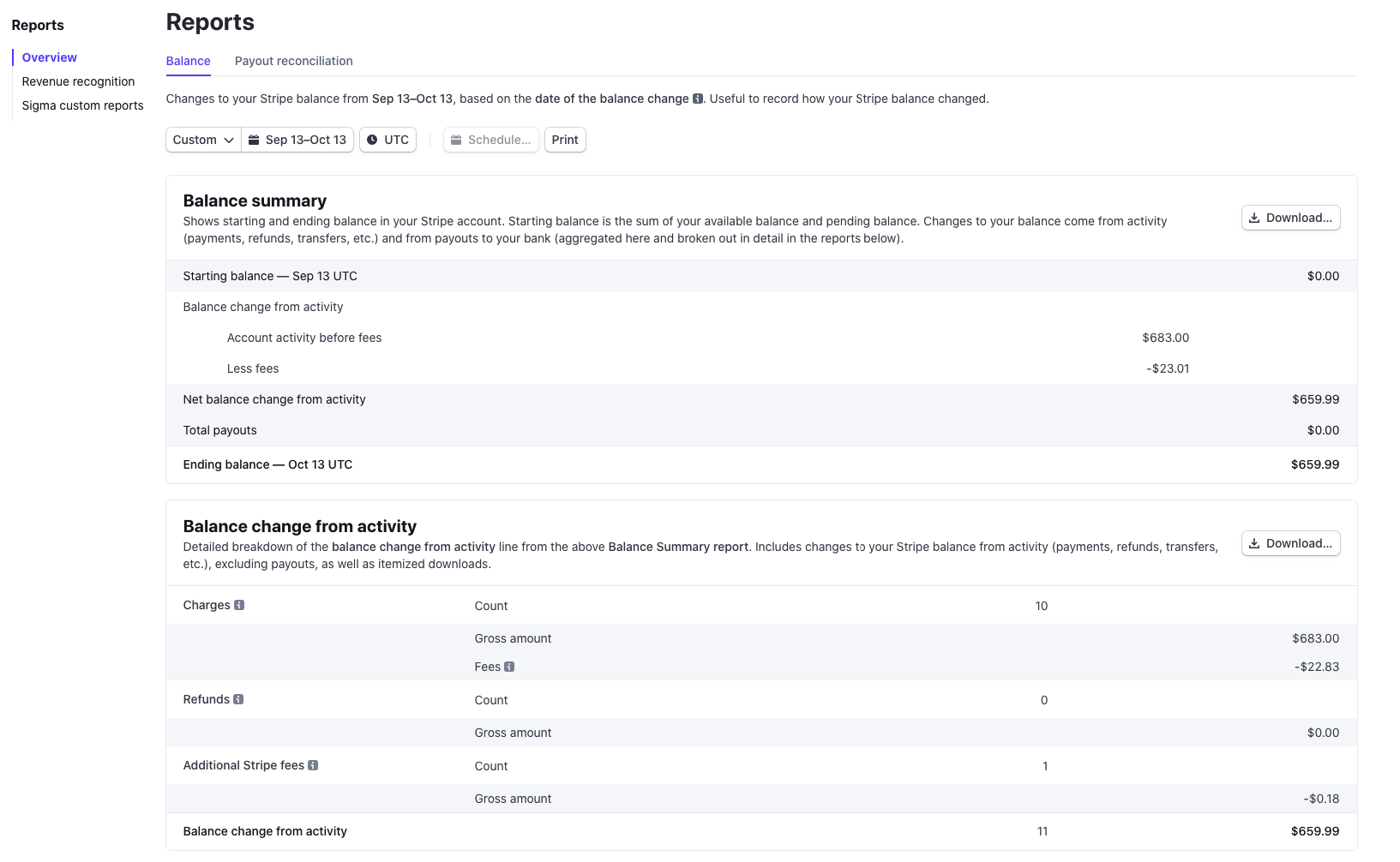In the image, detailed information is displayed with various text elements and graphical components. On the left side, in smaller black text, the word "Reports" is followed by a vertical line. Adjacent to the line, the word "Overview" appears in blue, alongside terms like "Revenue Recognition" and "Sigma Custom Reports."

Shifting our focus to the right side of the image, we see another instance of the word "Reports" in black text. Below this, the word "Balance" is prominently underlined in blue, which is followed by terms such as "Payout," "Reconciliation," and a detailed period descriptor, "Changes to your Stripe balance from September 13th - October 13th," based on the date of the balance change.

Beneath this section, the word "Custom" appears, accompanied by a downward-pointing arrow and the date range "September 13th - October 13th, UTC," with a square next to the word "Schedule." Below this grouping, in black text, there is a "Balance Summary" highlighted, which concludes with the amount of 683.

Additionally, the section denotes "Late Fees" or "Less Fees," amounting to a negative value of -23.61, leading to a final ending balance of 659.99. Further down, the image presents a section titled "Balance Change from Activity," featuring subcategories such as "Charges," "Refunds," "Additional Stripe Fees," and again, "Balance Change from Activity."